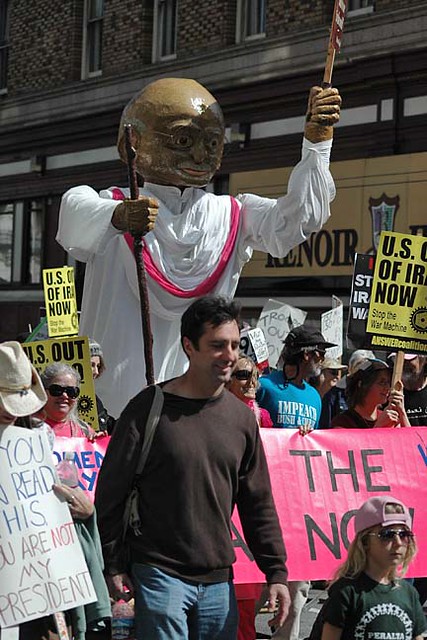The photograph captures a vivid scene from a lively protest or demonstration. At the forefront stands a young white man in a dark gray sweatshirt or Henley and faded jeans, beaming a bright smile. Beside him is a child sporting a pink baseball hat worn backward, sunglasses, and a short-sleeved gray shirt with a design on the front. The crowd, a diverse assemblage of people varying in age, gender, and race, is marching together, holding numerous signs. Some of the legible signs read, "U.S. out of Iraq now," and "If you can read this, you're not my president," while others are partially obscured. The protest unfolds on a bright sunny day, and many participants don sunglasses and hats.

A striking feature in the background is a towering puppet-like figure, possibly walking on stilts, dressed in white robes with a red sash, and holding a staff in one hand. The puppet has a large, sculpted greenish-gold head, adding a dramatic flair to the scene. The figure's left hand extends upward, though the object it holds is not visible. Behind the marchers, the backdrop includes a three-story building with light brownish bricks and stores on the lower levels, indicating an urban setting. The imagery is dynamic and rich, capturing the collective spirit and visual variety of the demonstration.